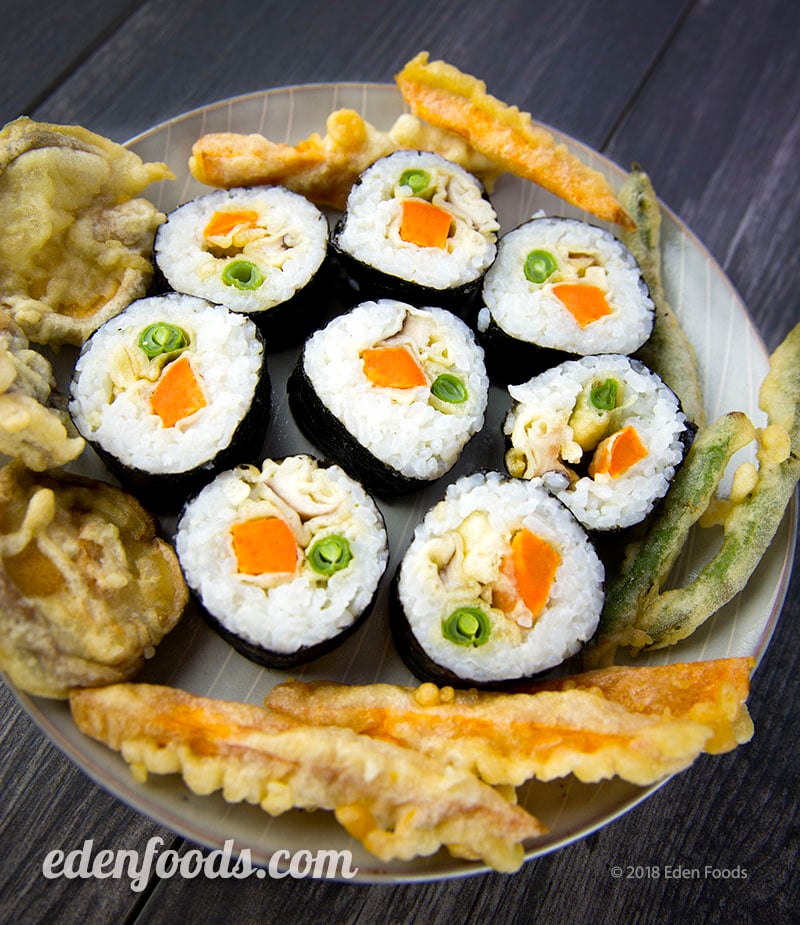The image captures a detailed top view of a visually appealing food presentation. Central to the photograph is an oval, gray plate adorned with white lines, resting on a flat wooden table. The centerpiece of the plate features eight meticulously arranged sushi rolls, possibly made of salmon, green onion, rice, and wrapped in seaweed. Surrounding the sushi are an assortment of tempura-fried items, including green beans, mushrooms, and leaves, adding a delightful variety of colors and textures to the dish. Contrary to one description, the plate is oval rather than round, and the table appears wooden rather than dark gray. The entire setting looks delicious and well-organized. At the bottom of the image, text reads "EdenFoods.com" along with a copyright mention, "2018 Eden Foods".